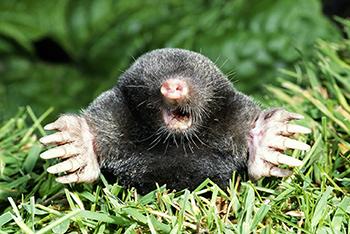The image features a mysterious, dark-furred creature resembling a mix between a mole and a groundhog, with a pink, pig-like snout. The animal is almost entirely black with barely-visible eyes, accentuated by prominent white whiskers. It has its mouth wide open, revealing teeth, and its formidable five-fingered front paws, each equipped with very long, sharp claws, are spread apart as if parting the thick, long green grass surrounding it. The creature's hands, almost skeletal in appearance, look menacing as they firmly plant on the grass. The background is blurred, showcasing an area likely filled with more grass or possibly leaves from trees or bushes, giving an overgrown, wild setting to the scene.